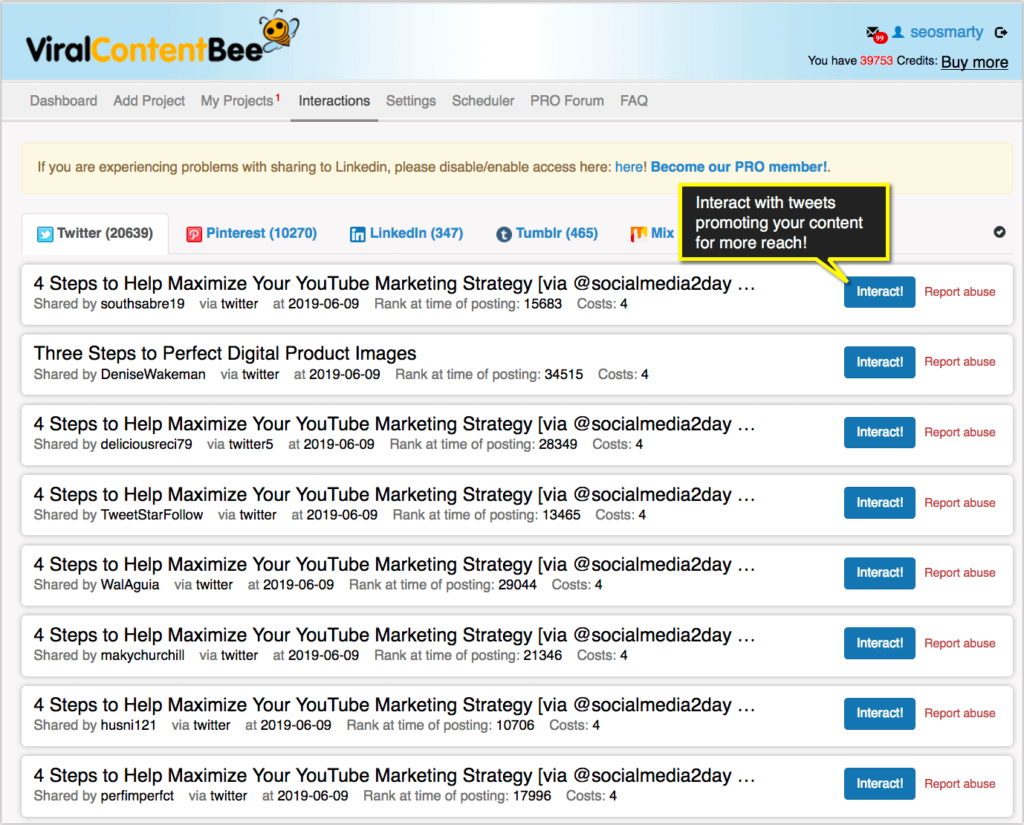Screenshot of the Viral Content B Website with User Interface Details and Interactions Tab

The screenshot displays the homepage of the website "Viral Content B." The website's name is creatively styled: "Viral" and "B" are in black font, while "Content" in the middle is yellow with black stripes, mimicking the appearance of a bee. An actual small bee icon is placed adjacent to the word "B."

In the upper right-hand corner, the username "seosmartie" is visible along with an inbox indicating 99 unread messages. The account has 39,753 credits, with an option to "buy more."

At the top of the page, a navigation menu includes the following options: Dashboard, Ad Project, My Projects (with a small notification indicating at least one pending project), Interactions, Settings, Scheduler, PRO Forum, and FAQ. The current tab is "Interactions."

A conspicuous yellow banner stretches across the screen, providing a notice about LinkedIn sharing issues and offering a clickable "here" link in blue to manage access. There's also a call to action in blue, encouraging users to become PRO members.

Below the banner, social media icons for Twitter, Pinterest, LinkedIn, Tumblr, and Mix are displayed, each accompanied by options available on their platforms. Notably, Tumblr has 20,639 options, Pinterest 10,270, LinkedIn 347, and Mix is slightly obscured by a black notification bubble that prompts users to "interact with tweets promoting your content for more reach." This bubble points to the interact button on one of the displayed options under Twitter.

Highlighted options include:
1. "Four Steps to Help Maximize Your YouTube Marketing Strategy."
2. "Three Steps to Perfect Digital Product Images."

Each option features an "Interact" button next to a "Report Abuse" button. The main focus on the screen is demonstrating the process of interacting with tweets to promote content for better reach.